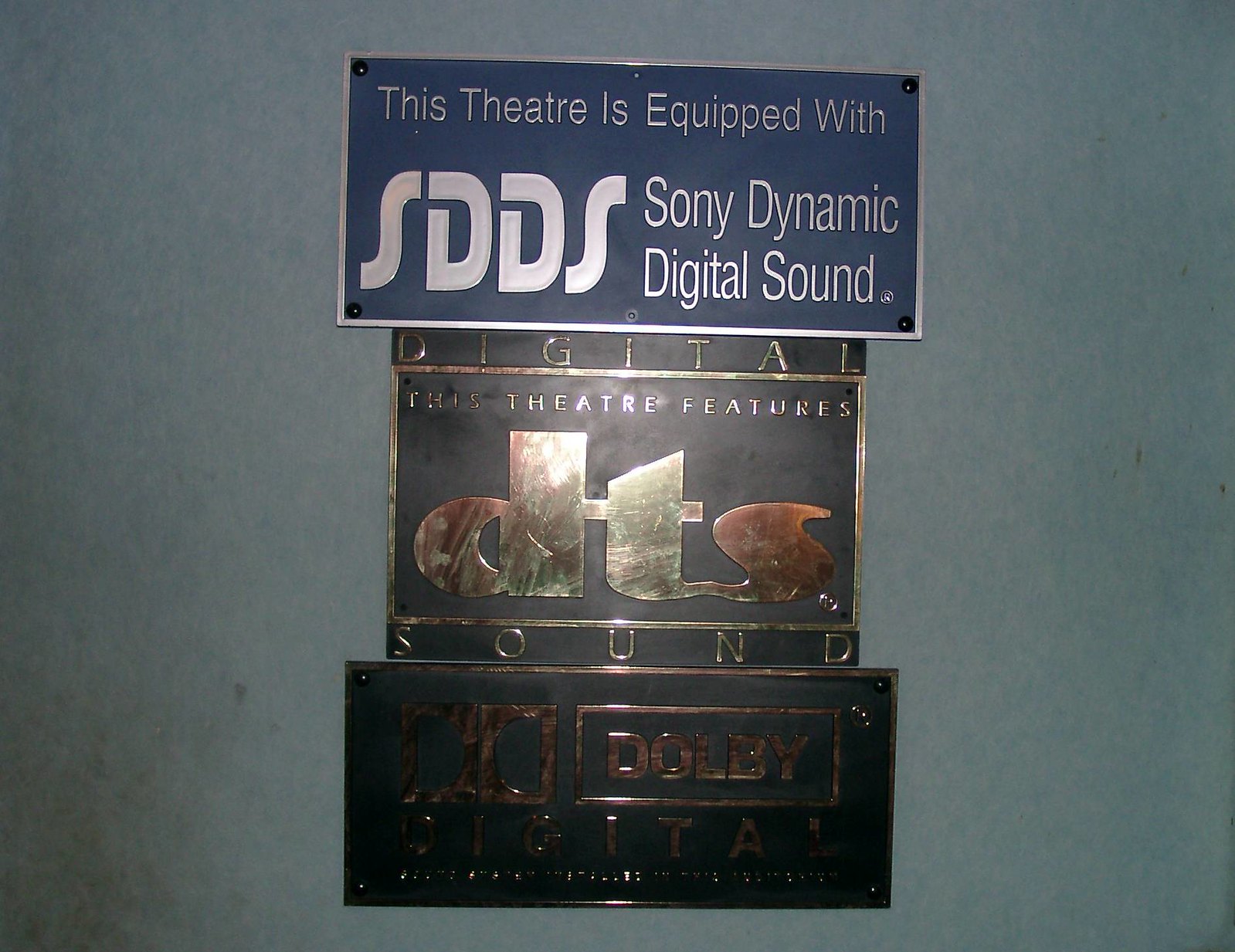The image depicts a series of three metallic plaques mounted on a slightly off-blue, steel-gray wall, each prominently displaying different logos or insignias associated with audio technologies commonly used in theaters. The top plaque is rectangular, featuring a navy blue background with silver lettering and a silver outline, stating "This theater is equipped with SDDS, Sony Dynamic Digital Sound" in large, eye-catching letters. Below it, a bronze-colored plaque with a black background and gold lettering reads, "Digital, This Theater Features DTS Sound," with the text equally pronounced. The bottom plaque, darker with a copper hue and copper outline, showcases the Dolby Digital logo and text, including the iconic Dolby "DD" symbol. These signs are aligned vertically, highlighting the exceptional sound equipment the theater boasts, creating a promise of an enhanced movie-watching experience for its patrons.